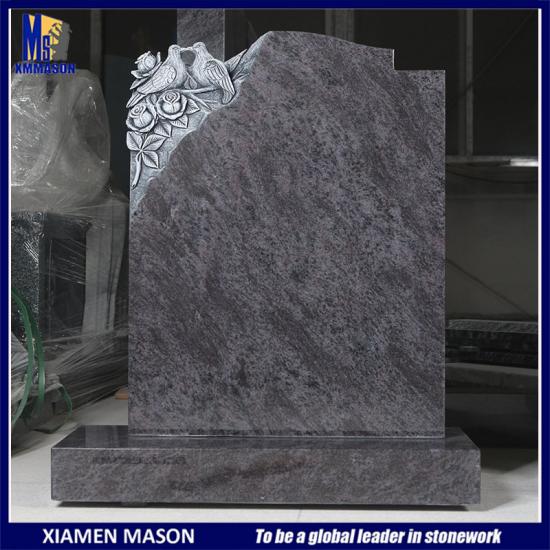This rectangular image, slightly taller than it is wide, features a blue border. At the bottom, it displays the text "Xiamen Mason to be a global leader in stonework" in white. The central focus of the image is a shiny gray marble tombstone with a simple design. The tombstone has an intricate engraving of two lovebirds nestled among roses and leaves in the top left corner, almost sculpted to protrude from the stone. The tombstone sits on a flat base and is presented against a background of varying dark gray shades, which remain indistinct. At the top left corner of the image, there is a logo that reads "MS Xiamen Mason." The overall presentation suggests the image could be an advertisement or a mock-up for stonework craftsmanship.